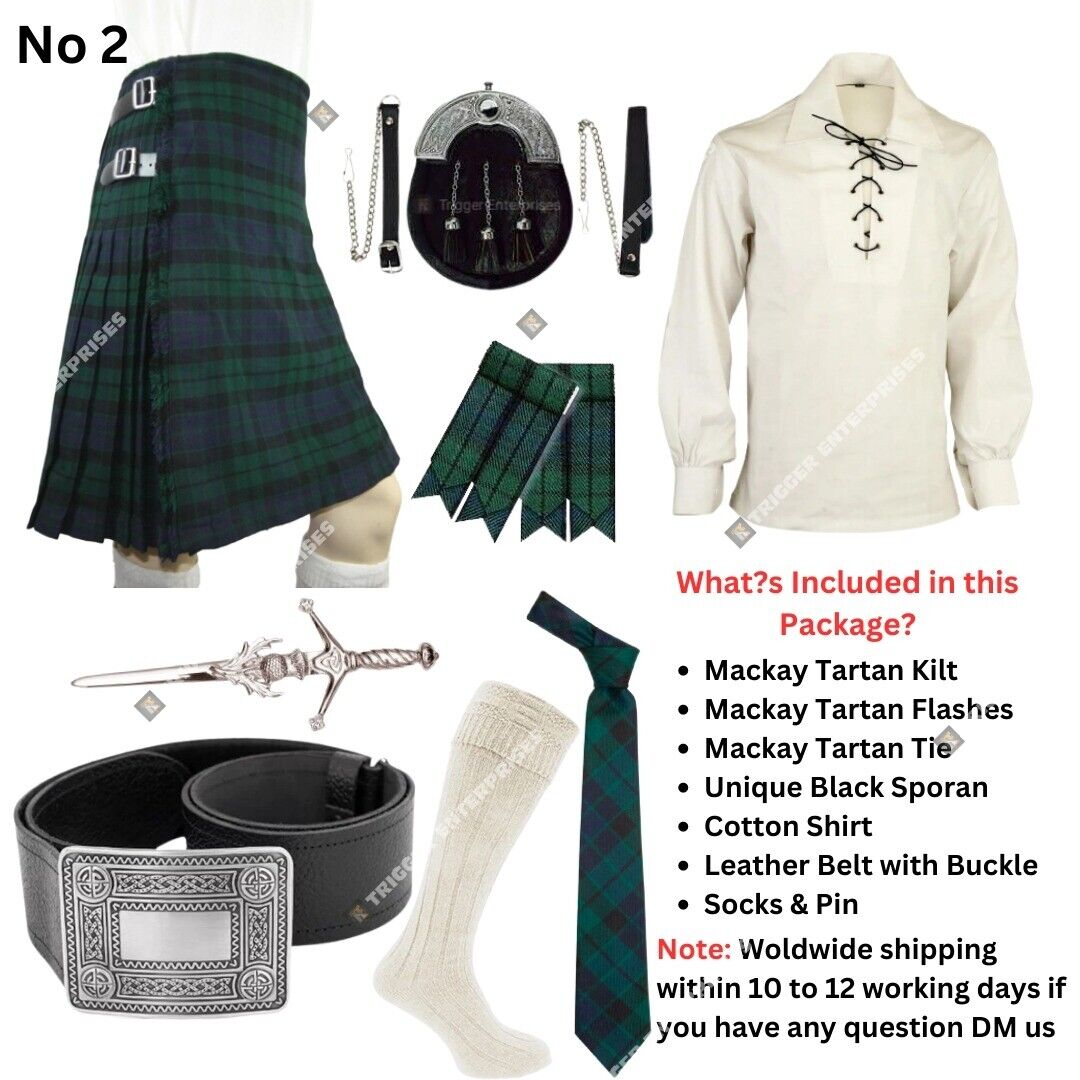This is a detailed advertisement for a premium Halloween costume set, presented as a catalogue page. The top left corner of the page prominently displays the number "2." The main image features a torso dressed in a McKay Tartan kilt paired with knee-high white socks. Accompanying the kilt is a unique black sporran. 

Adjacent to this are visuals of a long-sleeved white cotton shirt with a lace-up front, a matching McKay Tartan tie, and a sample of the fabric used. The inclusion of a black leather belt with an ornate silver buckle and a small dagger adds to the outfit's authenticity. Further, there's a clear, concise text in the bottom right corner specifying, "What's included in this package": McKay Tartan Kilt, McKay Tartan Flashes, McKay Tartan Tie, Unique Black Sporran, Cotton Shirt, Leather Belt with Buckle, Socks, and Pin. Below this, in red, there's a shipping note: "Worldwide shipping within 10 to 12 working days. If you have any questions, DM us." A watermark for Trigger Enterprises subtly covers part of the image, ensuring brand authenticity.